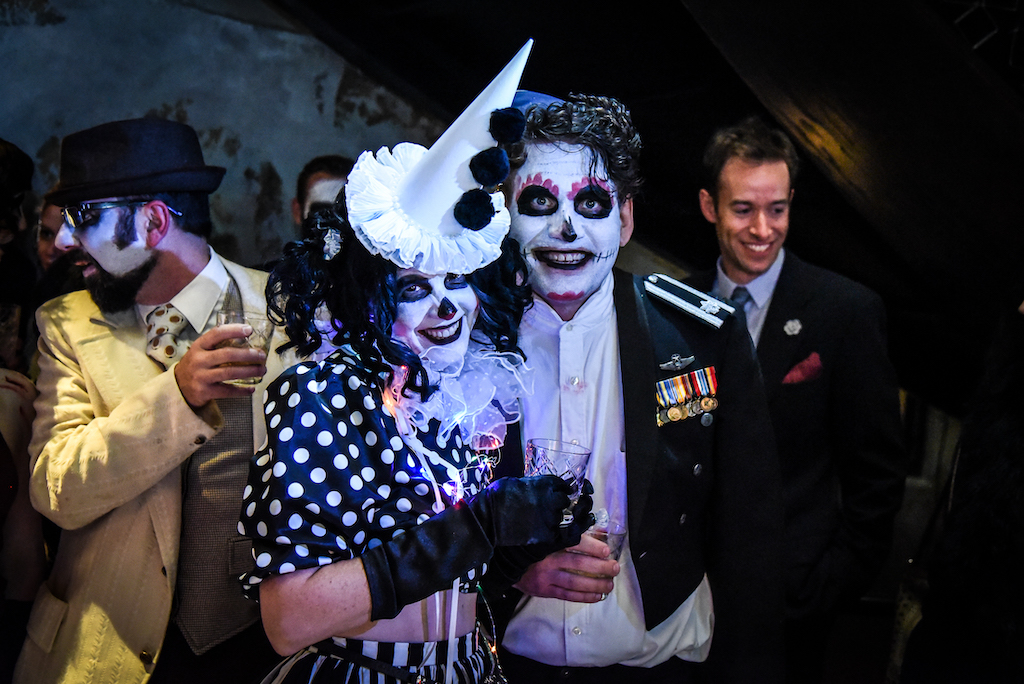This image appears to capture a lively dress-up or Halloween party, possibly themed around the Day of the Dead. Central to the scene are a couple standing in the foreground, both with curly black hair and white and black face paint that includes black circles around their eyes and pink details. They're smiling, clearly enjoying the festivities.

The woman, positioned on the left, is adorned in a striking outfit featuring a pointed white hat with black ornaments, a black dress covered in white polka dots, and long black gloves. She also sports a lace collar and ruffles around her face, carrying a drink that seems to be in a plastic cup. Her companion, on the right, dons a white shirt under a black jacket, reminiscent of a military uniform, complete with colorful decorations and medals on the chest. He holds a similar drink to hers.

In the background, there are several other individuals, including one man in the far left turned to the side, wearing a white shirt, a khaki suit with a tie spotted with brown, black hat, and glasses, along with white and black face paint. Another man in a black suit without makeup stands behind the main couple. The entire scene is vibrant, filled with details that suggest a celebratory and festive atmosphere.